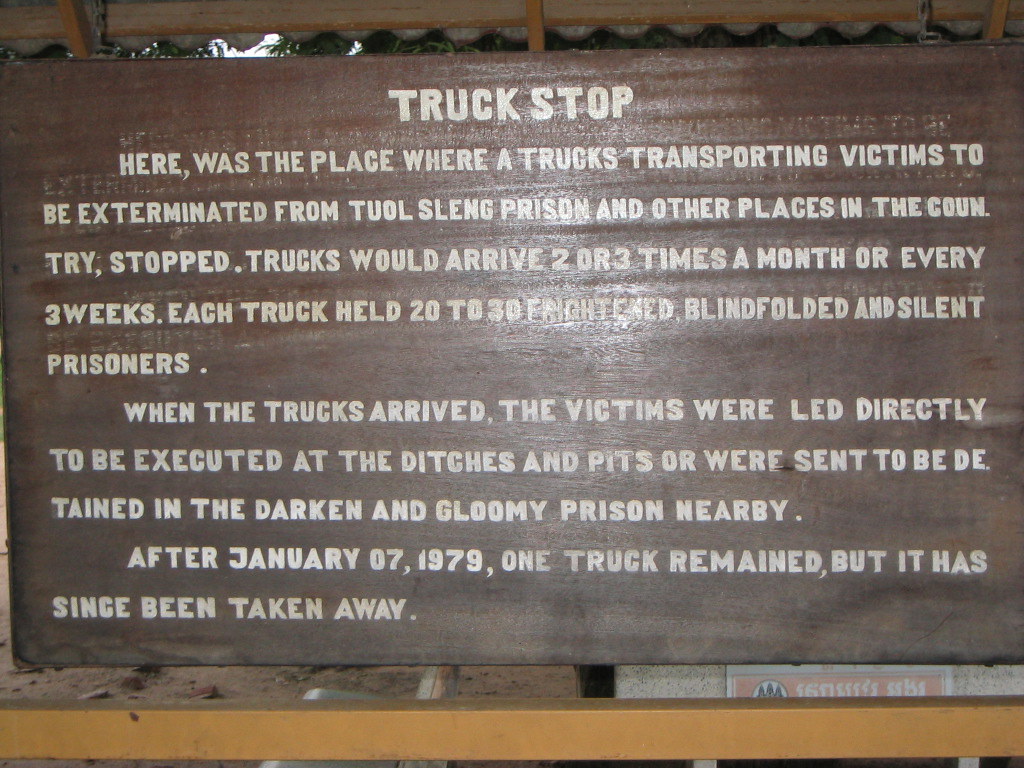This is an image of a large, brown wooden sign with off-white text that reads "Truck Stop" at the top. The sign, which appears to be mounted outdoors under the roof or awning of a tent-like structure, describes a historically significant and somber location. The inscription details the site where trucks transported victims destined for extermination from Tuol Sleng prison and other locations in the country. These trucks arrived two or three times a month, roughly every three weeks, each one carrying 20 to 30 frightened, blindfolded, and silent prisoners. Upon arrival, the victims were either executed immediately at nearby ditches and pits or detained in the dark, gloomy prison nearby. Notably, after January 7, 1979, one truck remained at this location, but it has since been removed. Additionally, the image shows a railing with vertical struts beneath the sign, suggesting the sign's placement in front of a walled structure. This memorial serves as a harrowing reminder of the atrocities committed and honors the memory of those who suffered and perished.